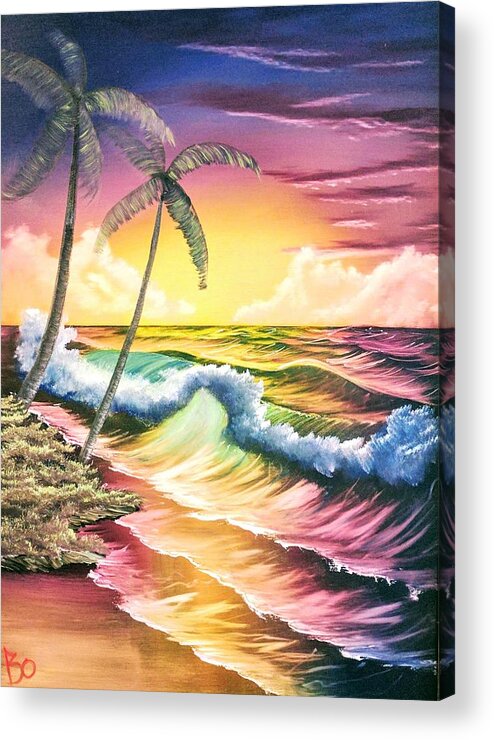This is a captivating, surreal painting of an ocean beach scene rendered in a spectrum of pastel colors. The ocean, situated on the right side, features waves crashing onto the sandy shore. These waves are a mesmerizing mix of pink, yellow, and light blue, with white foam cresting at the top. Beyond the lapping waves, the water continues in shades of yellow and pink interwoven with wisps of white. The sandy beach occupies the left side, exhibiting an unusual blend of yellow, pink, and brown hues. Near the shore’s edge, a patch of white, gray, and black foliage grows, from which two tall palm trees emerge, one thicker and taller than the other. The trunks and leaves of these palms are detailed in shades of gray and white. A vibrant sky stretches above, starting with a yellow glow likely from the fading sun, encircled by pink tones, giving way to a royal blue that gradually darkens towards the top. Wisps of white and purple clouds are scattered across the sky, particularly concentrated towards the right. In the distance, white clouds hover on the horizon, accentuating the ethereal yellow glow beneath them. On the bottom left corner of this arresting painting, the letters "BO" are written in red, enhancing its mystique.